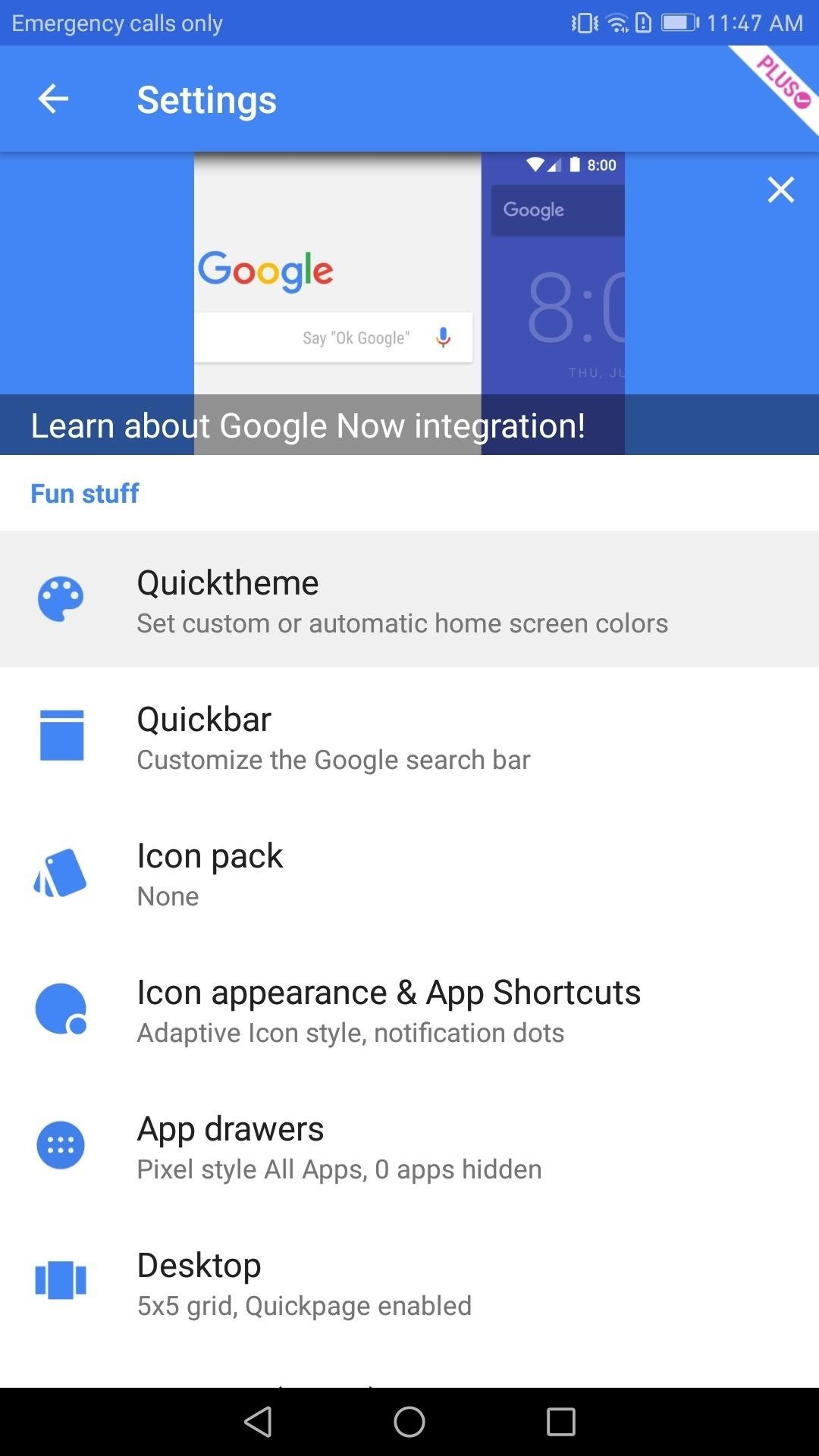The image is a mobile screenshot of a settings page, captured at 11:47 a.m. The status bar at the top indicates "Emergency calls only," suggesting the bill may be unpaid. Below the status bar, there's a blue header with white lettering saying "Settings." Just beneath this header is another blue rectangle containing what appears to be a screenshot of a Google search page. Overlaid on this is a small interstitial message stating "Learn about Google Now integration."

In the main body of the settings page, a white background features blue icons and black text. At the very top of this section is a blue heading labeled "Fun Stuff." Below this heading are several options listed with corresponding icons to their left:

1. Quick Theme
2. Quick Bar
3. Icon Pack
4. Icon Appearance
5. App Shortcuts
6. App Drawers
7. Desktop

At the bottom of the screen, the standard navigation icons for back, home, and recent apps are visible.